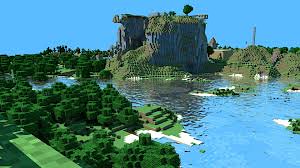This is a small, detailed screenshot of a Minecraft landscape, suggesting a game environment with blocky aesthetics. The focal point of the scene is a picturesque lagoon, surrounded by verdant green trees and grasslands. There’s a notable structure resembling medieval castle ruins, with only two walls standing and no ceiling, adding a sense of historical intrigue. Amidst the vivid green flora, there are light patches of moss or grass, accentuating the terrain's texture. A striking geological feature sits prominently in the middle — a large, imposing rock formation, possibly with a tree on top. In the water, tiny white islands or pads dot the surface, adding to the scene's complexity. The sky above is a clear, brilliant blue, perfectly reflecting in the similarly blue water below. Off in the distance, a white tower stands out against the horizon, contributing to the tranquil yet enigmatic atmosphere of this digital landscape.